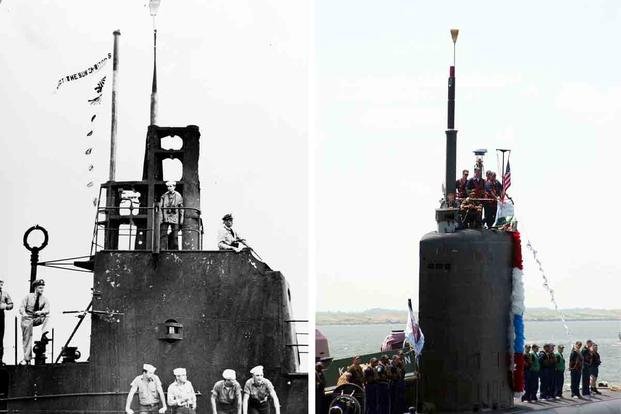This image consists of two panels showing the top view of a naval vessel. The left panel, in black and white, features a group of sailors and officers on the deck. The sailors sport white sailor hats, light-colored t-shirts or shirts with rolled-up sleeves, and darker pants. Among the seven visible figures, two are dressed in brown uniforms with black ties and officer's caps. Prominently, a steel mast or pedestal rises from the vessel's deck.

The right panel offers a color perspective of a likely similar, if not the same, vessel from a different angle. This view reveals red, white, and blue decorations adorning the ship, hinting at a celebratory or ceremonial event. A white flag with darker hues is partially visible. The crew in this image wears dark clothing and baseball-style caps, though details about them are less discernible. Both images highlight the presence of the steel pedestal, a defining feature of the ship's structure.